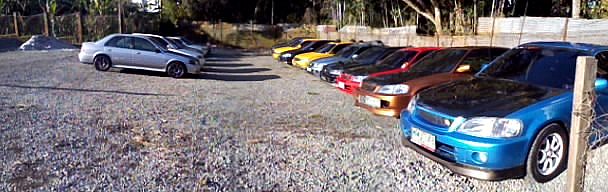In the foreground of this outdoor photograph, multiple cars are parked in a gravel parking lot. The right side of the image features a longer row of cars backed in at a slight angle, facing inwards to the left. This row includes a striking sequence of colors: a blue car, followed by a gold car, a red car, a black car, a silver car, a yellow car, another black car, and another yellow car, with a gap between them. On the opposite side, there is a shorter row of mostly lighter-colored cars, including a few white and gray vehicles.

The background is framed by a combination of dark trees and fencing. In the upper left corner, a fence made of white material attached to vertical poles is visible. Further back, an elevated area with dry brownish grass, some green patches, and additional trees can be seen. A wooden post with attached chicken wire is positioned prominently in the foreground of the image. The overall scene depicts a typical gravel lot with an array of colorful sedans parked under the serene backdrop of nature and fencing.